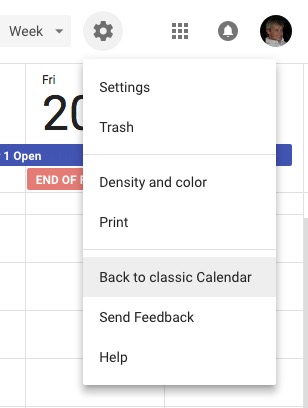The image is a screenshot of a calendar application interface with various elements displayed prominently. 

At the very top of the interface, there is a white background. In the top left-hand corner, there is a gray drop-down menu labeled "Week" in black text, accompanied by a small black upside-down triangle indicating additional selectable options. Next to this menu, there is a gray circular icon featuring a darker gray settings gear icon. It appears that this settings icon has been clicked, as a drop-down menu is visible.

The drop-down menu has a white background with black text. The options listed are:
1. Settings
2. Trash
3. Density and color (separated by a thin dark gray line)
4. Print
5. Back to classic calendar (another thin line separator)
6. Send feedback
7. Help

The "Back to classic calendar" option is highlighted in a grayish color.

To the right of the settings icon, there is an icon with nine gray boxes arranged in a 3x3 grid, forming a larger square. Further to the right, there is a dark circular icon with a white bell inside, presumably a notifications icon. On the far right, there is a circle-shaped avatar icon depicting a person with short grayish hair and a white collared shirt.

Below the top border, you can see a portion of the calendar interface. The top of the calendar displays the abbreviation "Fri" and the numbers "2" and "0," though the rest of the numbers are obscured by the settings drop-down menu. 

Beneath the date section, there is a blue horizontal rectangle spanning from left to right with the label "1, Open" on the left side. Directly underneath this blue rectangle, slightly to the right, there is a salmon-colored rectangular box with the partially obscured white text "End of something," also covered by the settings drop-down menu.

The calendar grid consists of large, long rectangular boxes with gray line separators. On the far right side of the interface, there is a gray scrollbar that appears to be scrolled all the way to the bottom.

Overall, the screenshot provides a detailed view of the calendar application's layout and user interface elements.